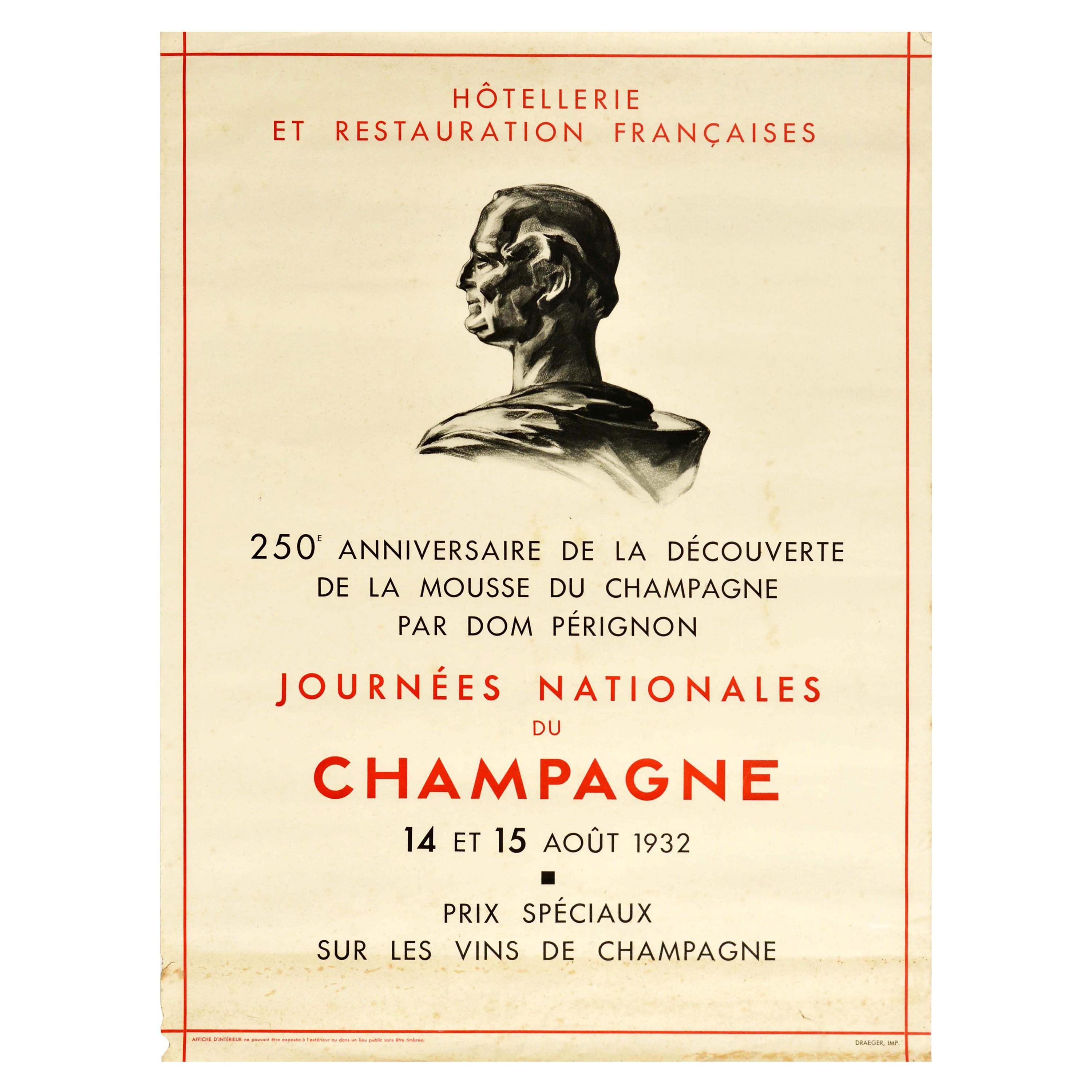This image appears to be a detailed illustration for a commemorative poster or label, possibly celebrating the 250th anniversary of a significant event related to champagne. The text, all in French, includes "Hotellerie et Restoration Française" at the top in red, suggesting an association with French hospitality and dining. The man depicted is an older individual, potentially in his 60s, dressed in robes or a coat with a hood; he is looking to the left. This image could be a drawing of a marble statue of this man. The background might resemble parchment paper, adding to the historical aesthetic. Key text in red includes "Journées Nationales du Champagne," emphasizing national celebrations related to champagne. Additional information notes the dates August 14th and 15th, 1932, and mentions "250th anniversary de la découverte de la mousse du champagne par Dom Pérignon," highlighting the discovery of champagne's effervescence by Dom Pérignon. The poster includes multiple sections of red and black text with red lines framing the entire page, tying together its celebratory and historical theme.